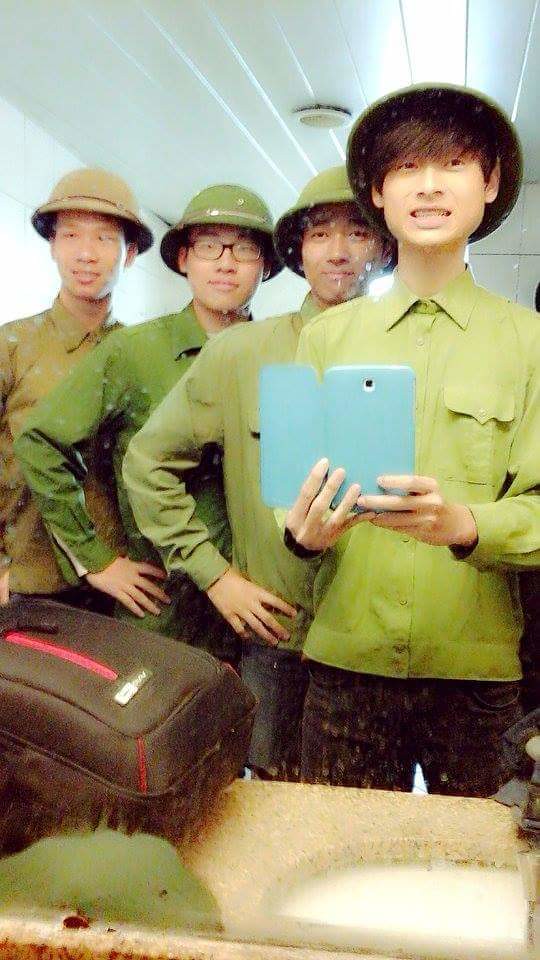In this indoor color photograph, we see a selfie taken in front of a mirror by four young Asian males, possibly Korean, Chinese, or Japanese, who appear to be around 18 or 19 years old. All of them are wearing military hats and long-sleeved military shirts in varying shades of green, except for the young man on the far left, who is wearing a brown hat. The first individual on the right is holding a blue smartphone with the camera icon visible, capturing the image. Each of the boys is smiling, with the one on the far right displaying a slightly open-mouthed, possibly awkward smile. The remaining three have smiles ranging from confident to tentative.

The mirror they are using to take the selfie shows signs of wear, with spots and residue indicating water splashes or toothpaste on it and a noticeable damage section at the bottom that obscures the view. The white ceiling above features a lined pattern and includes a visible smoke alarm or sprinkler. Below, a sink and counter are visible, with a black case lying on the left side of the countertop. The positioning of the boys starts with the one holding the phone closest to the camera, the second and third boys slightly to his left with their right shoulders visible, and the farthest left showing his torso and head. Despite the worn state of the mirror, the image captures a moment of camaraderie among the four young men.